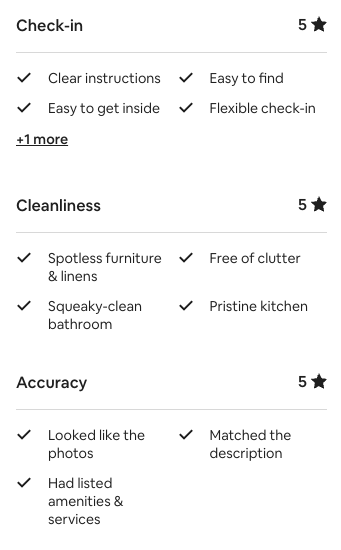This image depicts a check-in screen interface. In the upper left-hand corner, the word "Check-in" is prominently displayed in capitalized, black font. On the upper right-hand side, the number "5" is shown, accompanied by a black star immediately to its right. 

Directly below this, a thin gray separator line spans the width of the screen. The section below this line presents a review summary. The first row contains two items: "Clear instructions" and "Easy to find," each with a check mark to the left, indicating successful completion. The second row follows a similar format, listing "Easy to get inside" and "Flexible check-ins," both also marked with check marks on their left.

Beneath these rows, the text "1+ more" is underlined, suggesting additional items not fully visible in this section. The next section is dedicated to ratings, starting with "Cleanliness," which has been awarded five stars, followed by "Accuracy," also boasting a five-star rating.